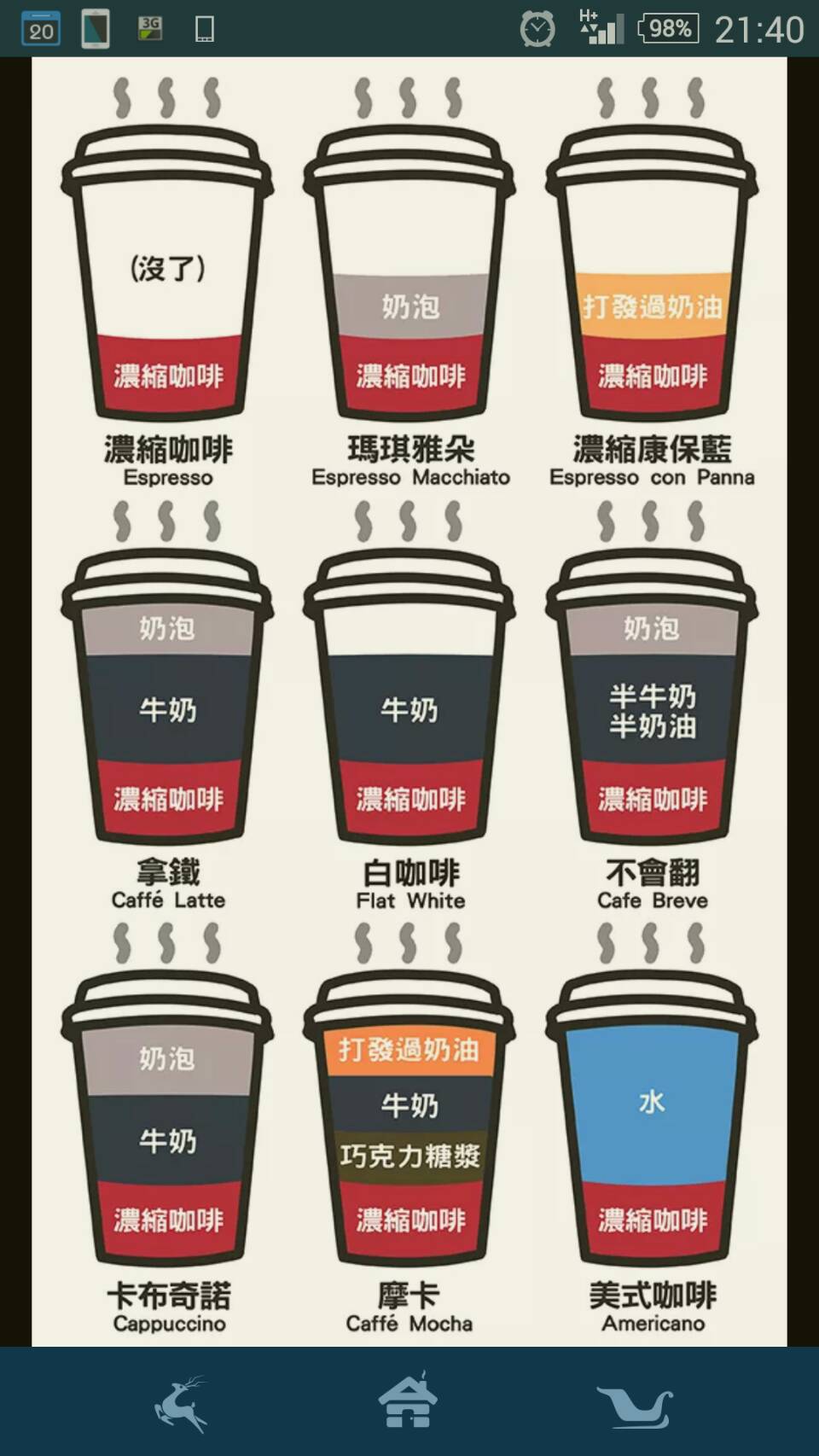This image is a screenshot captured on a smartphone, indicated by the black border around the screen displaying typical phone status indicators such as time (21:40), battery level (98%), signal strength (three bars), notifications, and other icons. The central image is a detailed poster illustrating nine different types of coffee, primarily labeled in what appears to be Chinese or another Southeast Asian language, with accompanying English text for each coffee type. The beverages are as follows: Espresso, Espresso Macchiato, Espresso Con Panna, Café Latte, Flat White, Café Breve, Cappuccino, Café Mocha, and Americano. Each coffee is depicted in a cup with varying color bands—red, black, gray, yellow, orange, and blue—that delineate the differences in coffee composition. Steam lines above each cup signify that they are hot drinks. The cups are meticulously arranged, showing diverse color schemes and layers that visually indicate the specific makeup of each coffee type.